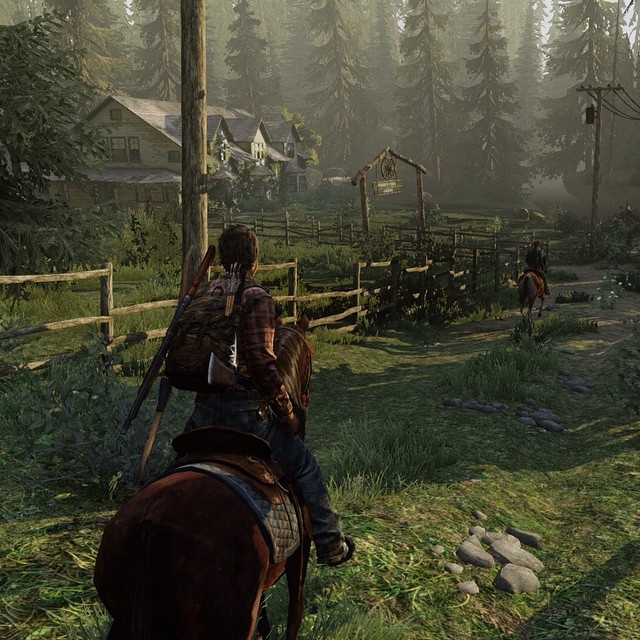The image appears to be a detailed painting, possibly mistaken for a screenshot from a computer game, depicting an enchanting woodland scene. Prominently, in the upper left corner, a light-colored, two-story house stands at an angle. The house features windows on its upper level and arched entryways on the ground floor, complemented by a wraparound porch. Extending from the house is a wooden fence that borders lush, green grass, adding to the serene ambiance.

In the lower left of the composition, a person rides away from the viewer on a brown horse. The rider, who appears to be carrying a bow and arrow on their back, guides the horse towards the house. Both the horse and rider are facing away, creating a sense of movement and direction in the scene. The backdrop is a forest of towering evergreen trees, their dense foliage casting intricate shadows across the verdant landscape. The interplay of light and shadow contributes to the painting's depth and realism, enhancing the overall immersive quality of the woodland setting.